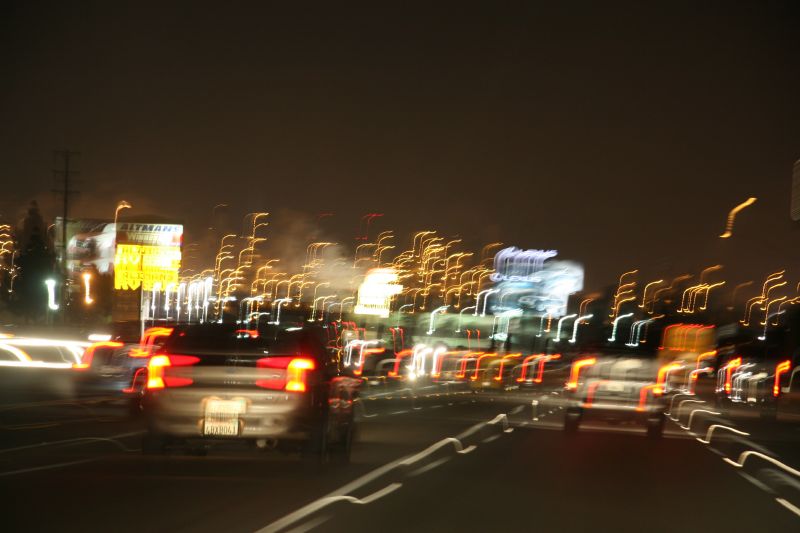This is a very blurry photograph taken at night from a car driving along a freeway, depicting perhaps three or four lanes of traffic. The car from which the photo is taken is in the third lane from the left. Directly ahead, there is a blurry car with motion-blurred brake lights, and to the left, there is another vehicle. In the furthest left lane, there's another car visible. The image has been purposely distorted to create light trails, with all the lights—brake lights, streetlights—forming streaks and contrails that curve around to the right. The night sky is dark, gradually fading to a lighter brown towards the city lights, suggesting a clear sky with no clouds. In the background, tall buildings glow, contributing to the cityscape. On the left edge of the freeway are billboards, which appear more stable compared to the motion blur of the cars. Beside the billboards, a completely black silhouette of a pine tree and a telephone pole are visible. The overall feeling is one of fast movement, with all the elements in the photo emphasizing a sense of speed and dynamic motion.